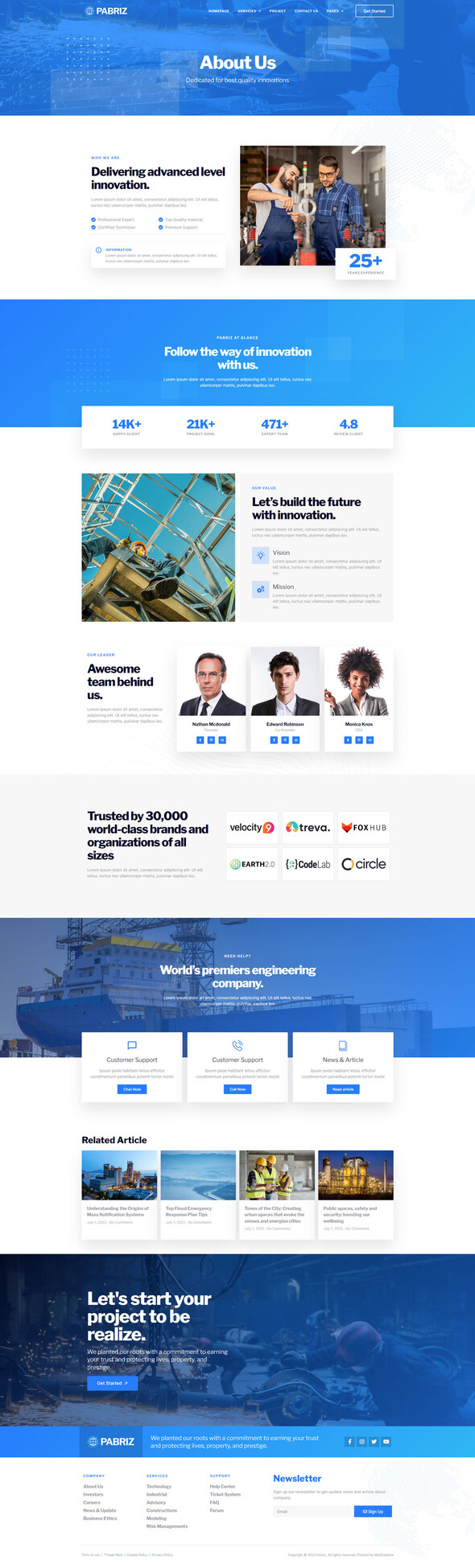This screenshot from the Purpris website showcases its dedication to delivering high-quality innovation. The website employs a sleek design using a blend of white, blue, and black colors. Specifically, white text is used against blue backgrounds, while black text contrasts with white backgrounds. At the top, the website's name "Purpris" is clearly displayed.

In the central section of the screenshot, there is an image depicting two men, presumably builders or engineers, working diligently side by side in what appears to be a workshop. Their experience spans more than 25 years.

Further down, the phrase "Let's build a future with innovation" is prominently highlighted as one of the company's slogans. The bottom portion of the screenshot showcases Purpris's international scope through images of massive ships, engineers wearing helmets, and a series of metal poles arranged adjacently. This powerful visual narrative emphasizes both the scale and the detail of the projects Purpris is involved in, underscoring their commitment to global innovation and engineering excellence.